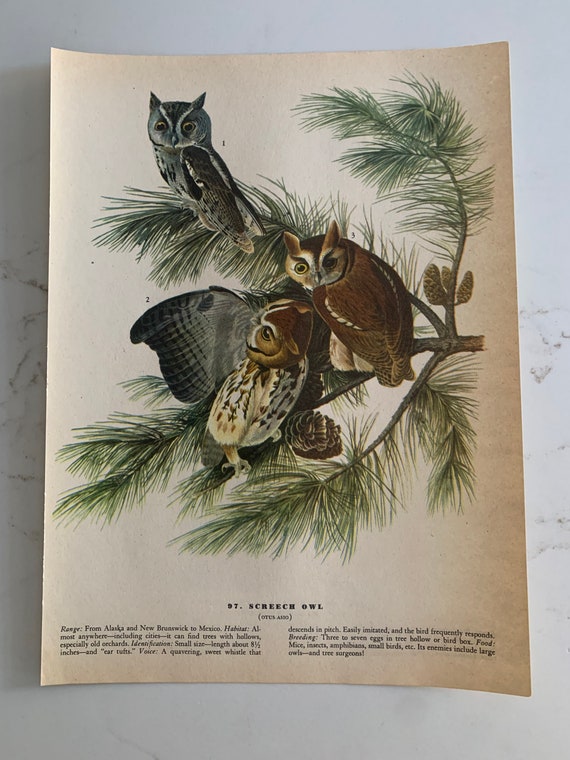The image is a detailed vintage drawing on brown paper, possibly a page taken from a book, depicting three Screech Owls perched on the fine, needle-like branches of a pine tree with three visible pine cones. At the top, a Gray Screech Owl with black or silver feathers perches prominently. Below, to the right, sits a Brown Screech Owl, while another Brown Screech Owl with a white, spotted chest perches at the bottom left, its head turned towards its open left wing. The drawing is highly detailed, accentuating their different feather colors and positions. At the bottom of the page, though small and largely illegible, the text provides detailed information about the Screech Owl, including their identification, habitat range from Alaska and New Brunswick to Mexico, diet, breeding habits, and natural enemies. The illustration vividly captures the intricate and diverse characteristics of these owls along with their serene natural setting.